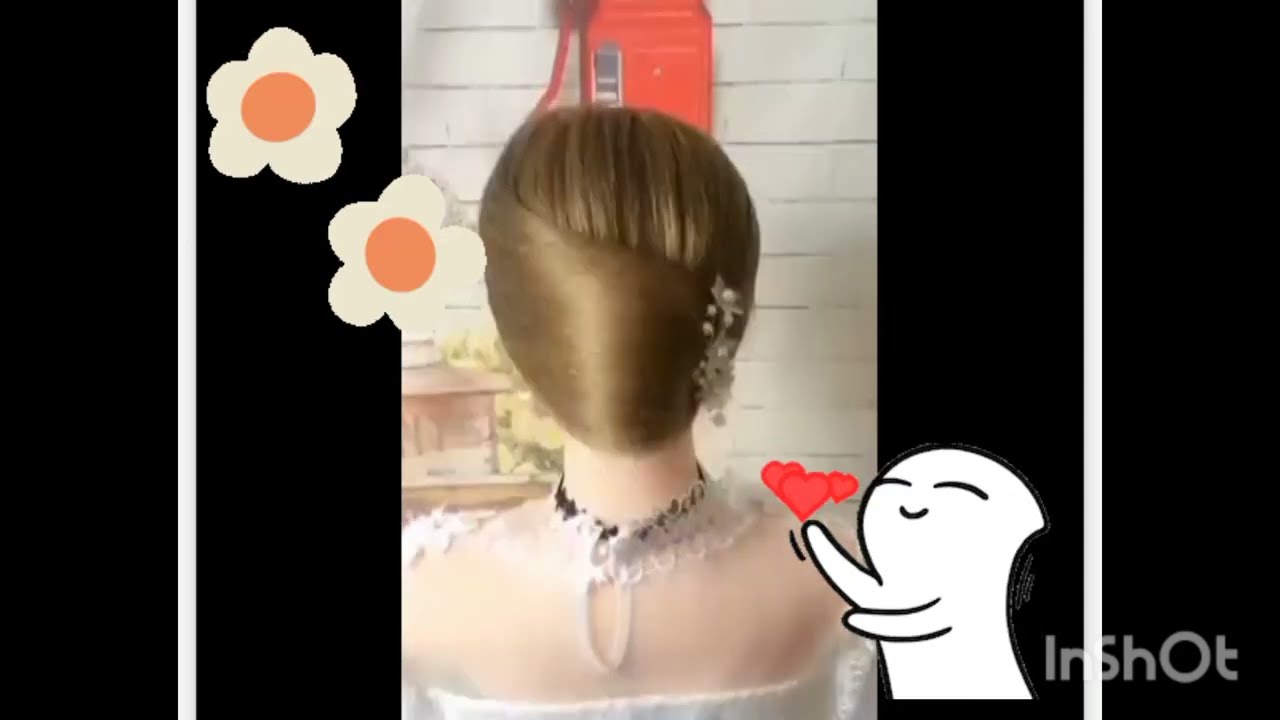The central image within a black-bordered horizontal rectangle features a woman viewed from behind, showcasing her in a seemingly bridal, white, lacy attire that includes a semi-transparent veil-like top. Her blondish-brown hair, tied neatly at the nape of her neck with a floral hairpin or similar accessory, is meticulously styled with no strands out of place. She is adorned with a black choker around her neck. This woman faces a white brick wall that displays a bright orange square or control panel in the center. Additionally, there appears to be a shelf with potential jewelry items to her left.

The image is elaborately edited with cartoonish graphics, including two white-petaled flowers with yellow centers in the upper left corner and a small, white, smiling creature in the bottom right. This creature is depicted holding a cluster of pink hearts. The bottom right corner also features the text "INSHOT" in grey letters, indicating the editing software used. The right and left thirds of the photograph are solid black with a thin white line separating them from the central image, creating a high-contrast framing effect. The predominant colors in the picture are black, white, brown, and orange.